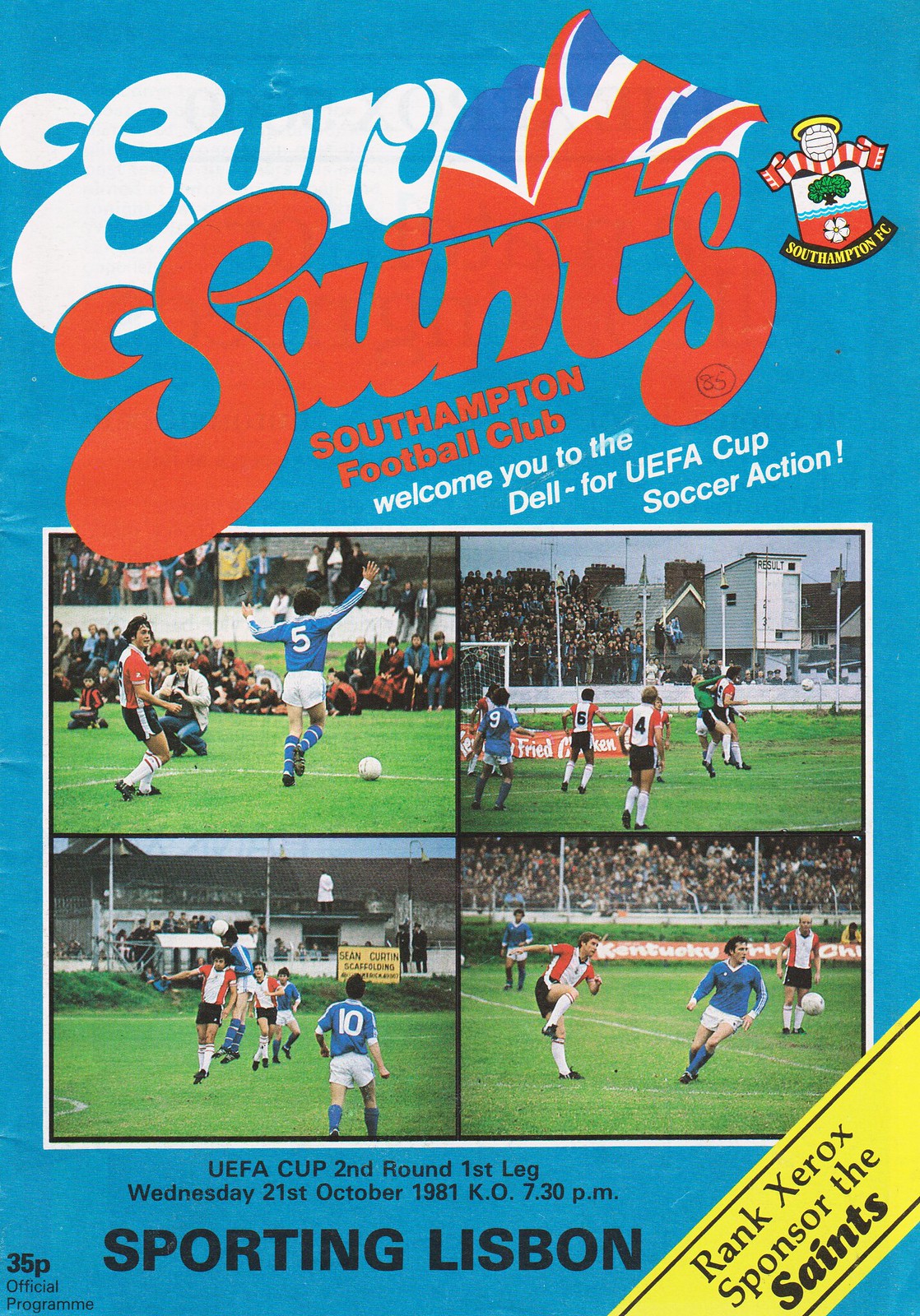The image is a vintage program cover from a sporting event, likely a magazine from 1981. The background of the cover is blue, with the title "Euro Saints" prominently displayed across the top third in white with an orange 'R'. Beneath that, it reads "Southampton Football Club welcomes you to the Dell for UEFA Cup soccer action". A stylized, rippled depiction of the Union Jack flag is included in the design. 

In the top corner, there is a Southampton FC logo. Below this, a rectangular section with four quadrants contains photographs of soccer matches, showing players in action, including notable visuals of players wearing numbers 5 and 10. At the bottom, the text details "UEFA Cup Second Round First Leg, Wednesday, 21st of October 1981, KO 7.30 p.m. Sporting Lisbon". Additionally, there is a yellow banner in the bottom right corner stating "Rank Xerox Sponsor of the Saints". The cover also mentions it is a "35 P official program".